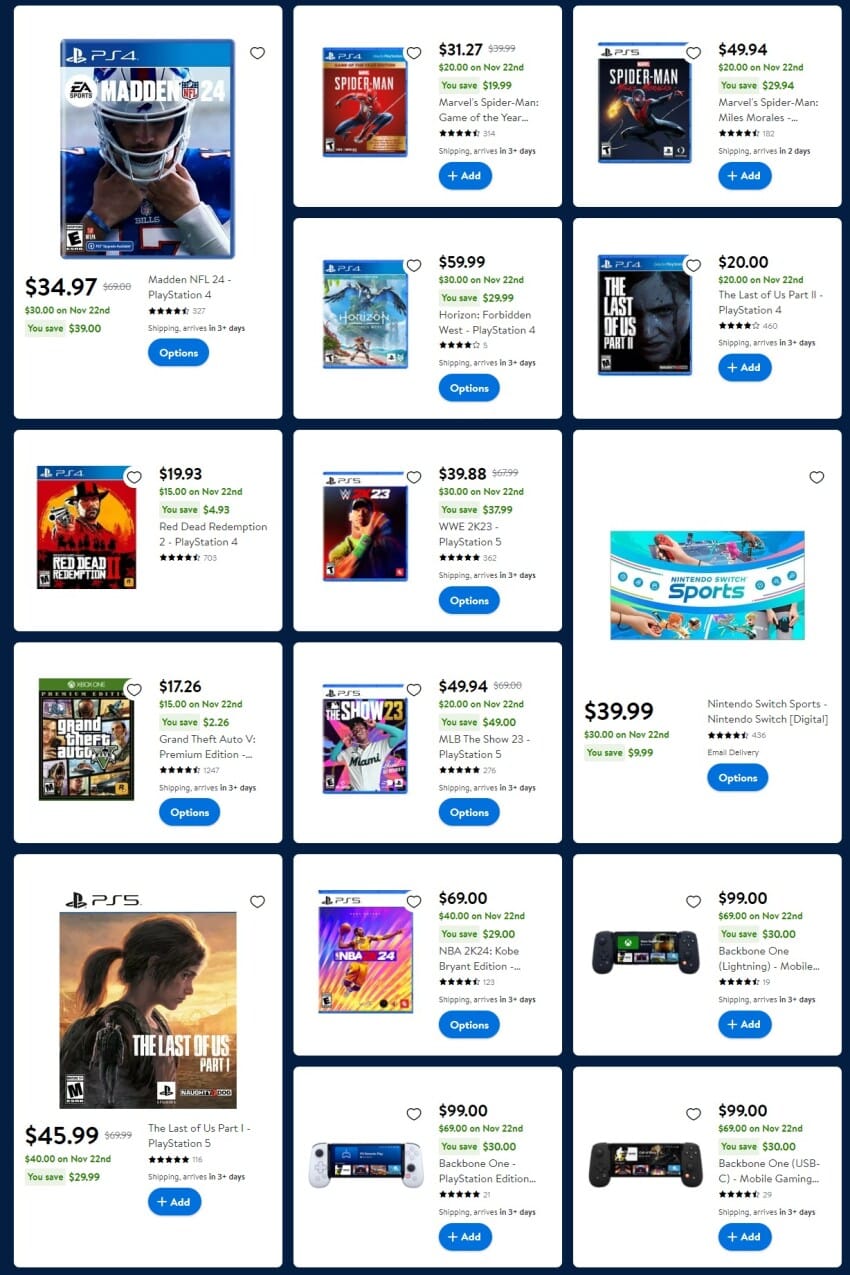Here is the detailed and cleaned-up caption:

---

The image displays a variety of video game cases and their corresponding prices. On the left, there is a "PS4 Madden" game priced at $34.97. To its right, a "Spider-Man" game case is marked at $31.27. Another blue "Spider-Man" game case is priced at $49.94. Next, "The Last of Us Part II" is listed at $20.00, followed by "Red Dead Redemption 2" for $19.93. There is also an unspecified item priced at $23.00. Another price of $39.98 is visible but not associated with a specific item.

"Grand Theft Auto V" is shown with a price of $17.26. Additionally, there is an item priced again at $23.00 and another at $49.94. A sports game is marked at $39.99. "The Last of Us Part I" is priced at $45.99. A "PS5" game is listed for $69.99.

The image also features controllers with screens, priced at $99.99 each. Out of the three controllers shown, two are black, and one is white.

---

This caption provides a detailed and organized description of the various items and their prices displayed in the image.